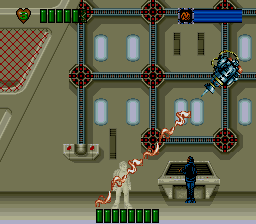This image is a detailed screenshot from a retro-styled video game, featuring an intricate scene with various elements. In the upper left-hand corner, there's a red heart icon with the number three inside, next to five green bars likely indicating health or energy. The background of the image is tan, overlaid with a grid formed by blue lines and marked by red circles at the corners, creating a squared pattern. The setting resembles a large laboratory or industrial factory with some white windows in the background. At the bottom, there's an off-white, ghostly or transparent character standing, while a figure in a blue outfit with his back turned appears to be operating a control panel. Diagonally above the off-white character, a robot is mounted on a set of tracks and is shooting a red, wavy laser-like flame towards the character. Additional details include six or seven green pill capsule-like objects at the very bottom, possibly representing another form of energy or power within the game.